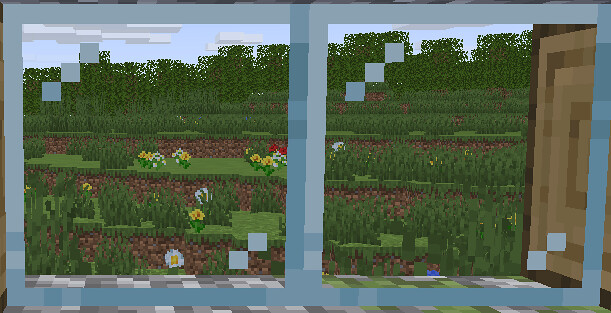This computer-generated image presents a visually cohesive stereoscopic view, divided into what appears as two parts but seamlessly connected in the center to form a singular, three-dimensional depiction. The left side of the image showcases an array of terraces adorned with vibrant flowers, creating a layered effect of cleared flower beds amidst additional floral arrangements. Green hedges provide a lush backdrop, enhancing the vibrant scene. Scattered bouquets of flowers nestle on the small, individual terraces, contributing to the rich textural variety.

In contrast, the right side of the image emphasizes the green background, showing more of the extensive hedges that frame the scene. Here, the terraces are less prevalent, focusing instead on the broader expanse of greenery. Intriguingly, a brown-on-brown square area encroaches from the right edge, resembling a door or a wall with a darker brown border, adding a touch of architectural intrigue. Together, these two perspectives—one abundant with floral terraces, the other dominated by verdant hedges and a subtle architectural element—merge to create a harmonious yet detailed stereoscopic image.